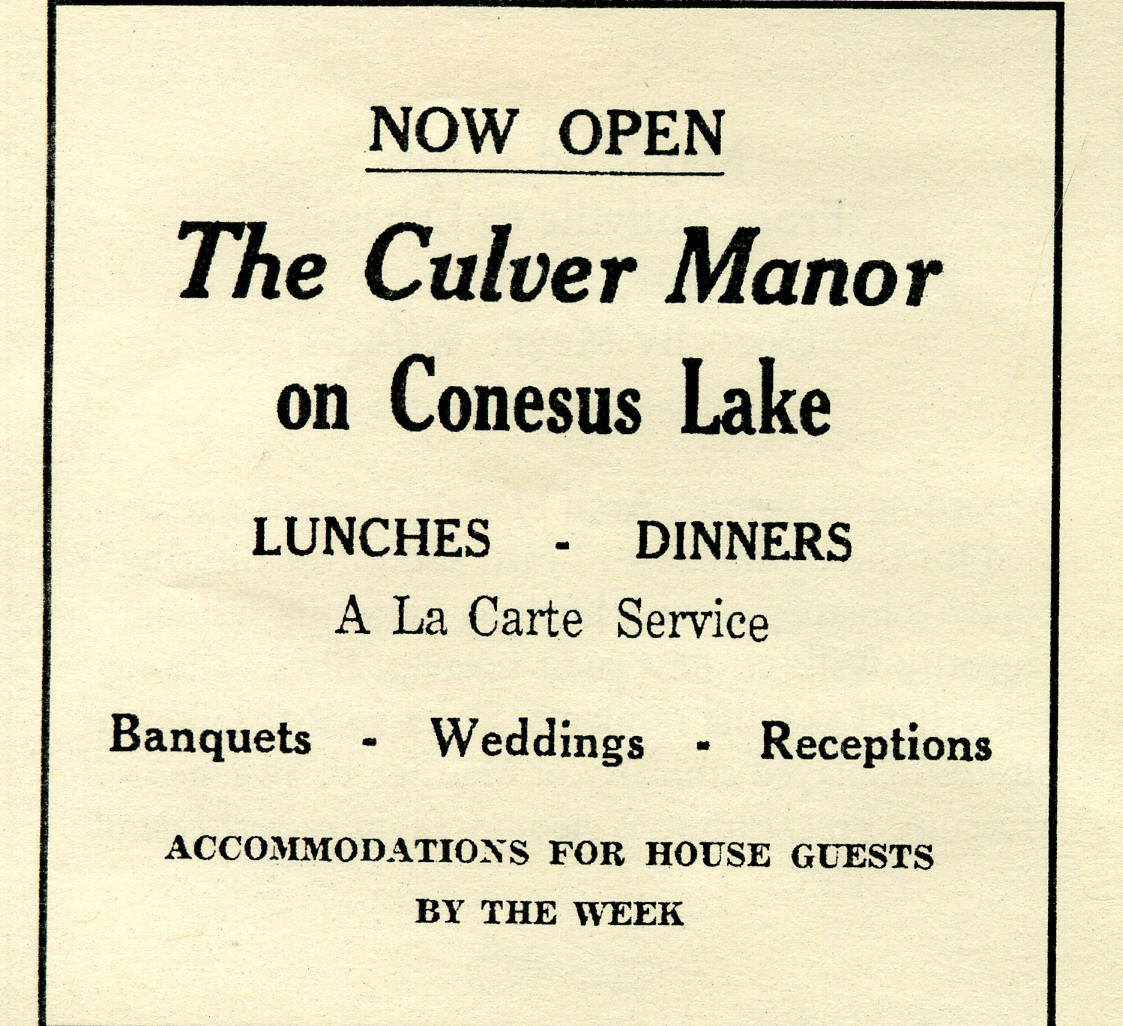This advertisement is presented on aging, cream-colored paper with a black border. Styled in a classic printing format, it exudes an antique charm. The headline, "NOW OPEN," is prominently displayed in bold, uppercase letters. Below this, "The Culver Manor on Conesus Lake" is showcased in elegant cursive and italicized text, creating a distinguished look. The subsequent lines list the services offered: "Lunches - Dinners - A la Carte Service" in slightly smaller type, followed by "Banquets - Weddings - Receptions" with only initial capitals. At the bottom, in the smallest font, it reads, "Accommodations for house guests by the week," all in uppercase. The overall composition suggests this piece was likely featured in a magazine or newspaper, adding to its vintage appeal.